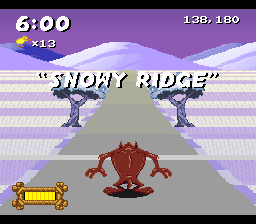The image is a snapshot from a pixelated, 16-bit style video game titled "Snowy Ridge," prominently displayed in white text at the center. The game appears to be displayed in a small, roughly square format, akin to a handheld console, bordered by thin horizontal letterbox strips at the top and bottom. 

In the center of the screen, we see a rear view of the Tasmanian Devil, a brown-furred cartoon character, standing on a straight gray path that extends into the distance. His arms are spread out to the side as if bracing against a fall, and his legs are splayed in a bow-legged stance. The path is lined with alternating horizontal stripes of white and purple, resembling snowy ridges. A pair of trees can be seen on either side of the path, just ahead of the character.

On the upper right corner of the screen, there are numerical indicators reading "138, 180," while the upper left corner shows a timer displaying "6:00". Below the timer, there is an icon of a duck or chick next to an "X" symbol followed by the number "13," potentially indicating lives or collectibles. The bottom left corner features a bar filled with golden blocks framed within a wooden pattern that vaguely resembles a wide skull shape. The overall color palette of the background is predominantly purple, emphasizing the snowy and cold theme of the game.